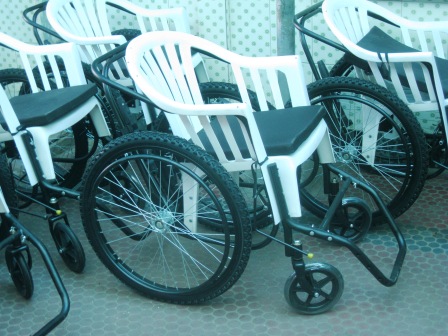The image depicts a collection of five modified wheelchairs, each constructed from plastic lawn chairs modified to function as mobility aids. The distinctive feature of these improvised wheelchairs includes their two large, bicycle-like black wheels accompanied by two smaller swiveling wheels for stability, which allow for maneuverability. The lawn chairs, which are white, serve as the seat and have been outfitted with thin dark green cushions for comfort. The metal framework, including the wheel handrails, appears to be either black or deep dark green tubing. A black bar is attached at the front of each chair, serving as a footrest. The wheelchairs are arranged such that one is prominently centered in the photograph while the others are positioned behind and to the sides of it. The setting of the photograph appears indoors, characterized by a floor with a subtle gray polka dot pattern. The background wall is white with blue dot accents, contributing to the overall bluish hue of the lighting in the scene.